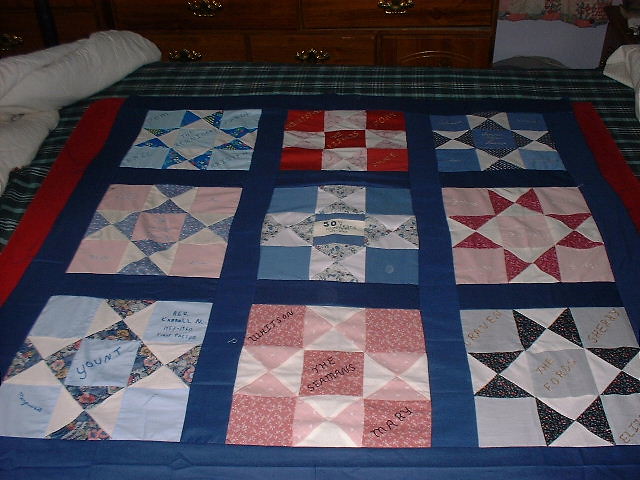This detailed photograph captures a small, patchwork quilt prominently displayed in the foreground, arranged on a bed with a plaid cover. The quilt is meticulously divided into nine sections, organized in a three-by-three grid. Each section features distinctive cross and diamond patterns, with additional rectangles or squares that highlight variations in the design. Notably, the quilt's vibrant color palette includes black and white, red and white, blue and white patches, and a pinkish-reddish hue. Each section is framed by blue fabric, providing a cohesive look.

The quilt is personalized with names in each section, suggesting it might be a family heirloom. "Yount," spelled y-o-u-n-t, can be seen prominently in one of the patches. In the background, the quilt is surrounded by various rolled-up or folded bedding items, forming a U-shape around it. Surrounding this setup, the bedroom scene includes a wooden chest of drawers, adding to the cozy, homely atmosphere of the image.